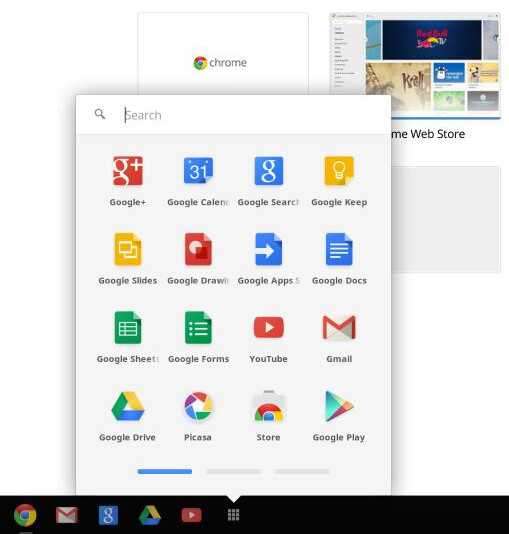A screenshot displays an operating platform window that appears to be a part of the Chrome Web Store on Google Chrome. The interface is likely running on an Android system, given the appearance and layout, which do not align with Apple's operating system. 

The foreground features a collection of Google apps icons on the left side of the screen, each vividly colored in Google's signature shades of blue, red, and yellow. The identified apps include Google Plus, Google Calendar, Google Search, Google Keep, Google Slides, Google Drawings, Google Apps, and Google Docs. Below these, green icons represent Google Sheets and Google Forms. Other app icons visible include YouTube, Gmail, Google Drive, Picasa, Google Store, and Google Play.

Towards the bottom of the screen, there are additional Google icons set against a black bar background: the Chrome icon, a generic Mail icon, another Google Search icon, the Google Drive icon, the YouTube icon, and the 'app grid' icon comprised of nine squares, which presumably opens the app window.

In the background of the app window, the Chrome logo and the word "Chrome" are distinctly visible. To the right, a partly cropped screenshot of the Chrome Web Store is shown, featuring a Red Bull advertisement and various colored icons, though the specific content is difficult to discern due to the cropping. The app window also covers another gray rectangle visible in the backdrop.